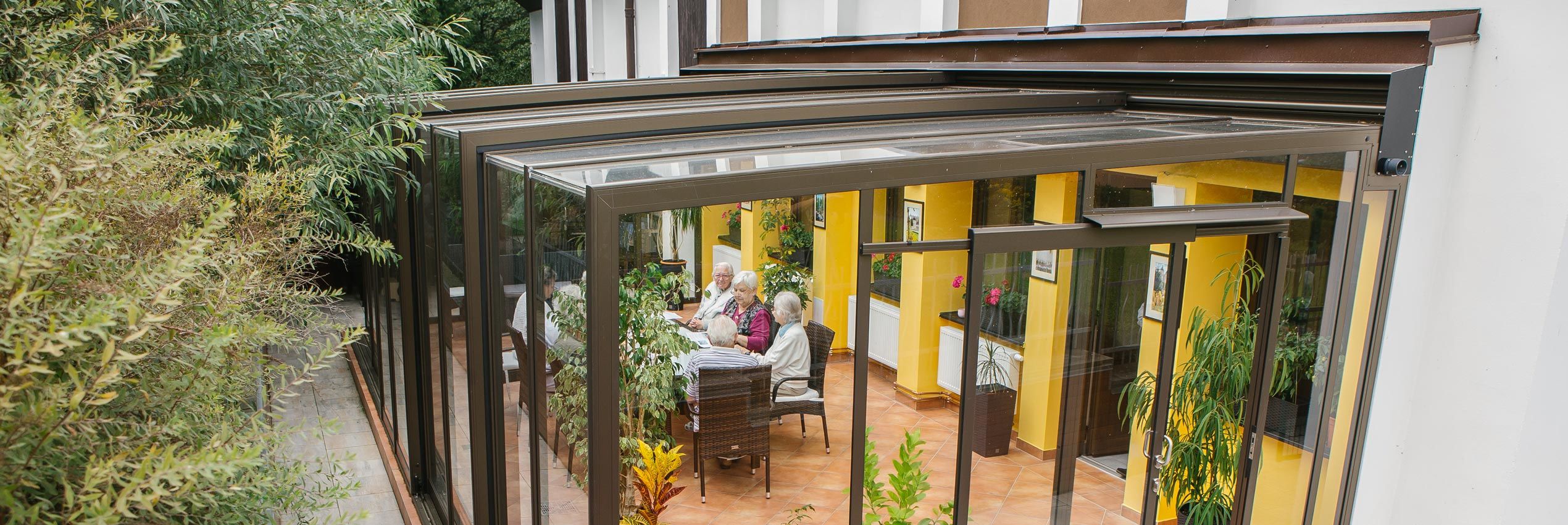This detailed photograph captures an outdoor setting adjacent to a restaurant, showcasing a harmonious blend of indoor and outdoor elements. The scene features a group of five elderly women, all with gray hair, gathered around a very long table within a sunroom-like glass enclosure. The building, divided visually by its yellow-painted lower half and white upper half, provides a charming backdrop. The women, adorned in modern clothing including white garments and a colorful blouse, seem to be engaged in a lively conversation while seated on brown chairs. 

Inside the glass-enclosed area, an array of lush houseplants and foliage creates a natural, inviting atmosphere, complemented by numerous windows that allow ample natural light to flood the space. Surrounding the glass enclosure are tall, verdant trees in varying shades of green, enhancing the picturesque and tranquil ambiance. This setting, characterized by its warm, welcoming appearance and rich plant life, exudes a peaceful, residential feel, making it an ideal spot for a daytime gathering or meeting.